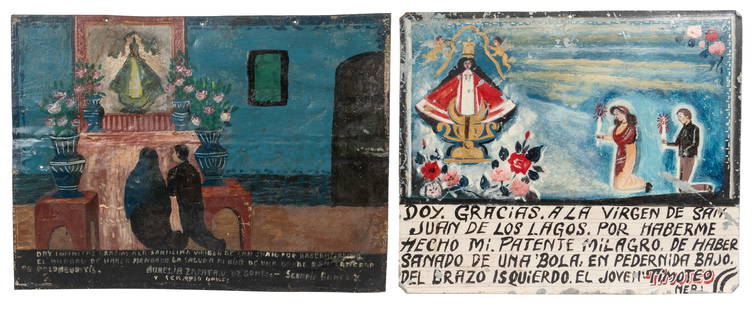The image depicts two antique artworks rich in religious symbolism. On the left, inside a blue-walled room with a brown floor, two individuals are kneeling in prayer, backs turned towards the viewer, facing an altar adorned with flowers and a framed image of a deity. The frame appears brown, and the painting it holds remains obscure, but it exudes a greenish hue. Surrounding the altar are tables with vases of flowers. A noticeable feature is a door leading out of the room. 

On the right, another religious artwork features text in Spanish and illustrates two people presenting offerings, including flowers, to a glowing deity surrounded by two cherubs. This scene also has a blue background and highlights a man and a woman holding white candles with burning yellow flames. The man is dressed in brown pants and a black shirt, while the woman wears a white dress with a red shawl. The painted strokes are loose, further enhancing the ethereal quality of the depicted spiritual ritual.